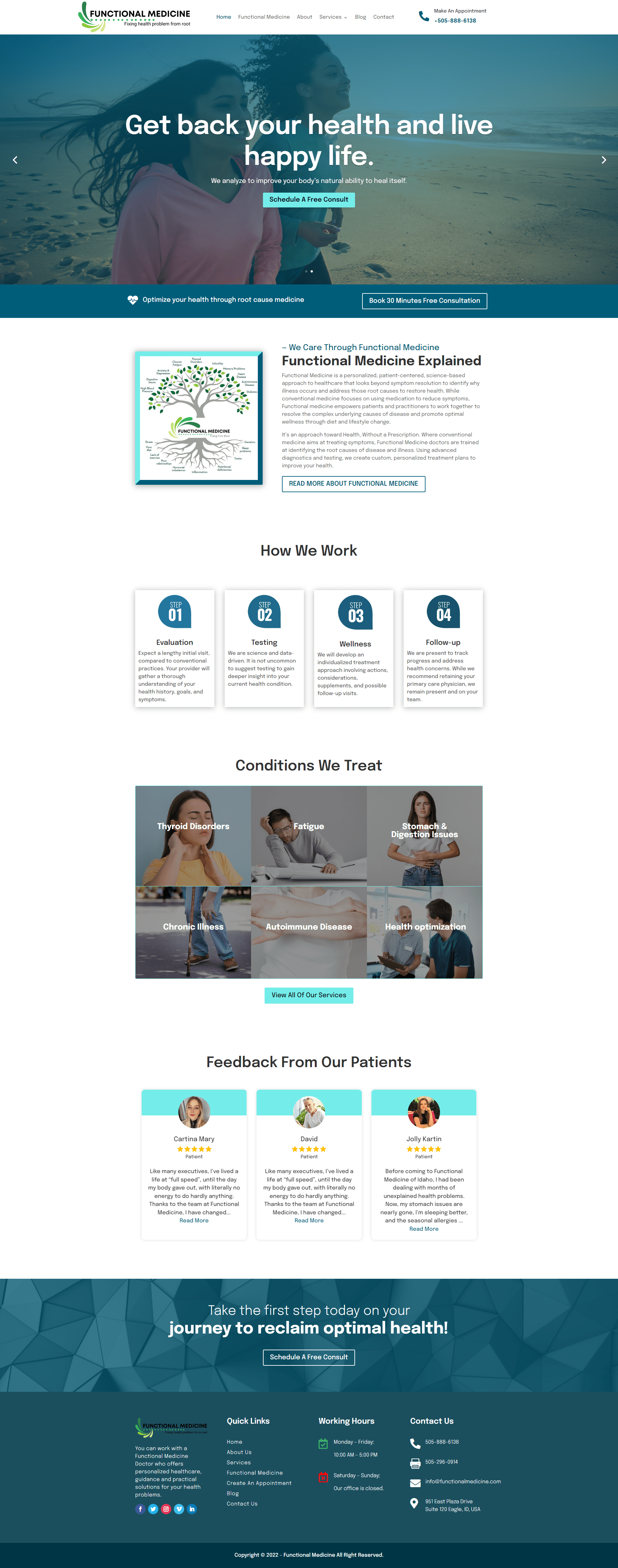The image is a vertical screenshot that appears to be taken from a phone, showcasing a website with a focus on health and wellness. At the very top of the screenshot, the website name and menu are present, though too small to be legible. Below this, a prominent image banner features two people running on the beach, overlaid with the text, "Get back your health and live a happy life." Beneath this slogan is a section of smaller text, accompanied by a noticeable blue button. Immediately below the banner is another section with tiny text.

Following this, on the left side of the screenshot, there is an image of a tree adjacent to some explanatory text. The text introduces the section titled "How We Work," which includes four distinct text boxes outlining different steps. Next, the section "Conditions We Treat" is displayed, featuring six images with descriptive white text overlays, and a prominent blue button beneath them.

Further down, the section "Feedback from Our Patients" showcases three testimonials, each accompanied by small profile images. The bottom of the screenshot features a blue background with the text "Journey to Reclaim Optimal Health" and several navigational links.